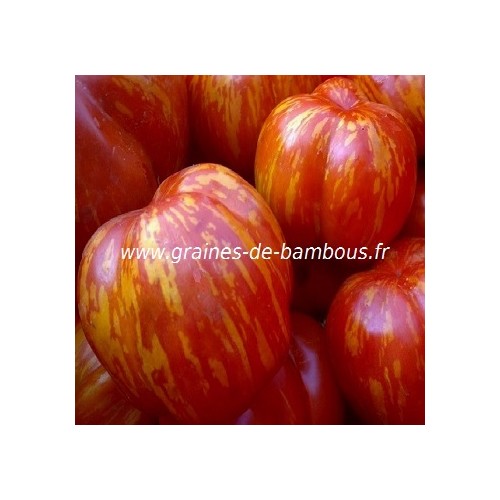The image showcases an assortment of bright red and yellow fruits or vegetables, possibly a mix of gourds or peppers, but the specific type is unclear. Dominating the center are two distinct specimens: one larger and fully visible with red and yellow hues, and another situated slightly behind it, also fully visible and similarly colored. Surrounding them are several partially visible fruits or vegetables, adding to a sense of abundance. The vivid colors—predominantly red with hints of orange and yellow—occupy the entire frame, creating a vibrant, almost sunlit atmosphere that suggests the picture was taken outdoors, perhaps at a market. Across the large central fruit, white lettering spells out "www.granus-d-bambos.fr." The background items appear slightly blurred, emphasizing the central focus on the two main fruits or vegetables. The objects are stacked, possibly indicating they are displayed for sale. Overall, the image presents a bright, colorful, and lively scene.